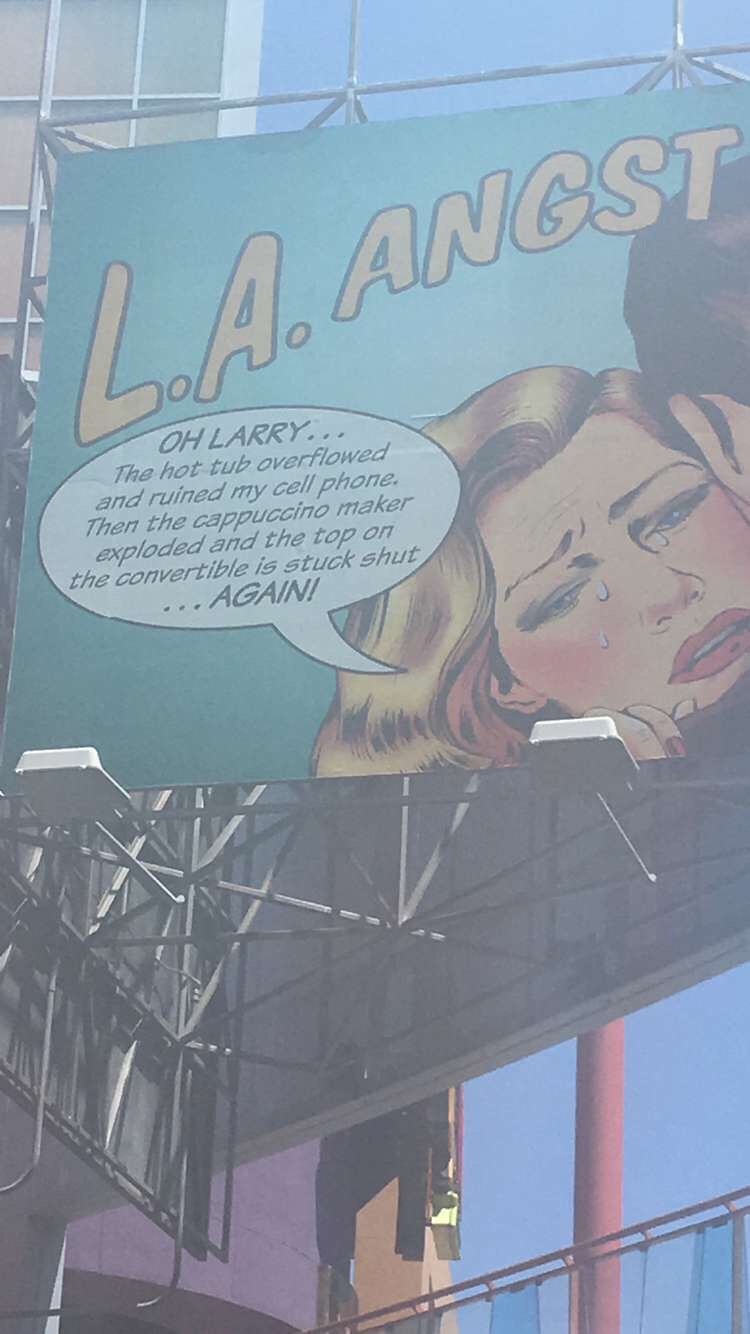The image is a photograph of a billboard taken outside against a blue sky. The billboard, mounted on a wire metal beam frame, has a greenish background on the visible left portion, giving it a hazy appearance due to the lighting. At the top of the sign, yellow letters spell out "L.A. Angst." Below this, in a white speech bubble with black text, it reads, "Oh Larry, the hot tub overflowed and ruined my cell phone, then the cappuccino maker exploded and the top on the convertible is stuck shut again!" 

A cartoon-style woman with long, straight, wavy blonde hair and full red lips is depicted on the right side of the billboard, with a couple of tears dripping down her face, emphasizing her distressed expression. The comic-style artwork and dramatic narrative suggest a humorous take on the misadventures typically associated with Los Angeles life.